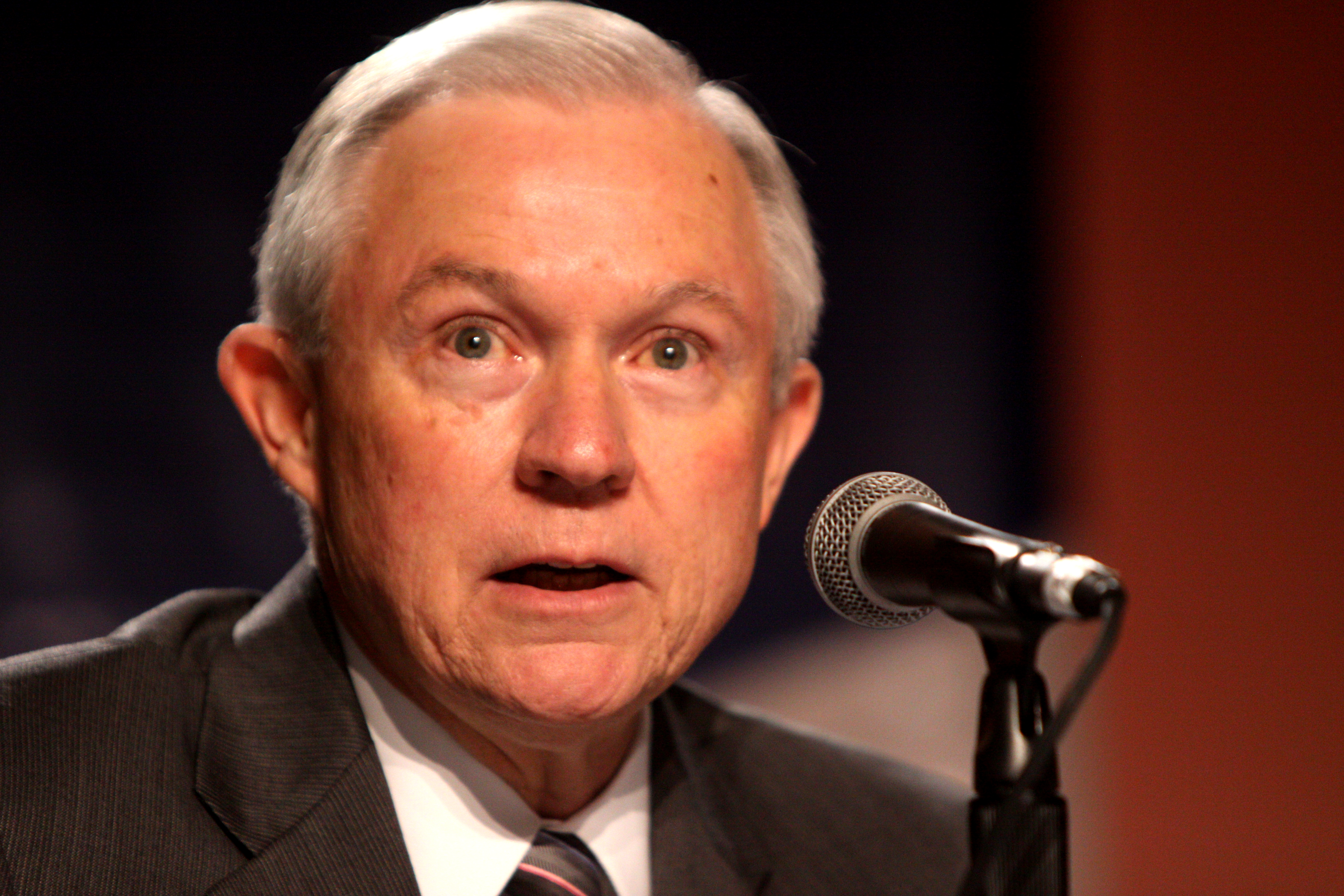This image captures an older man, likely a politician or public figure, speaking into a microphone. The man appears to be in his 60s or 70s, with short, slicked-back gray hair and a clean-shaven face. His eyes are greenish, and he has a few moles or birthmarks on his face. Dressed in a gray or brown sports coat with a white shirt underneath, he wears a distinctive tie featuring black material with diagonal pink and possibly blue stripes. The microphone in front of him is a classic model with a black body and a silver mesh top, mounted on a stand with a visible cord extending from the back. The background is out of focus but shows elements of blues, browns, and possibly a curtain. The man is speaking, as indicated by his open mouth and the engaged expression on his face.